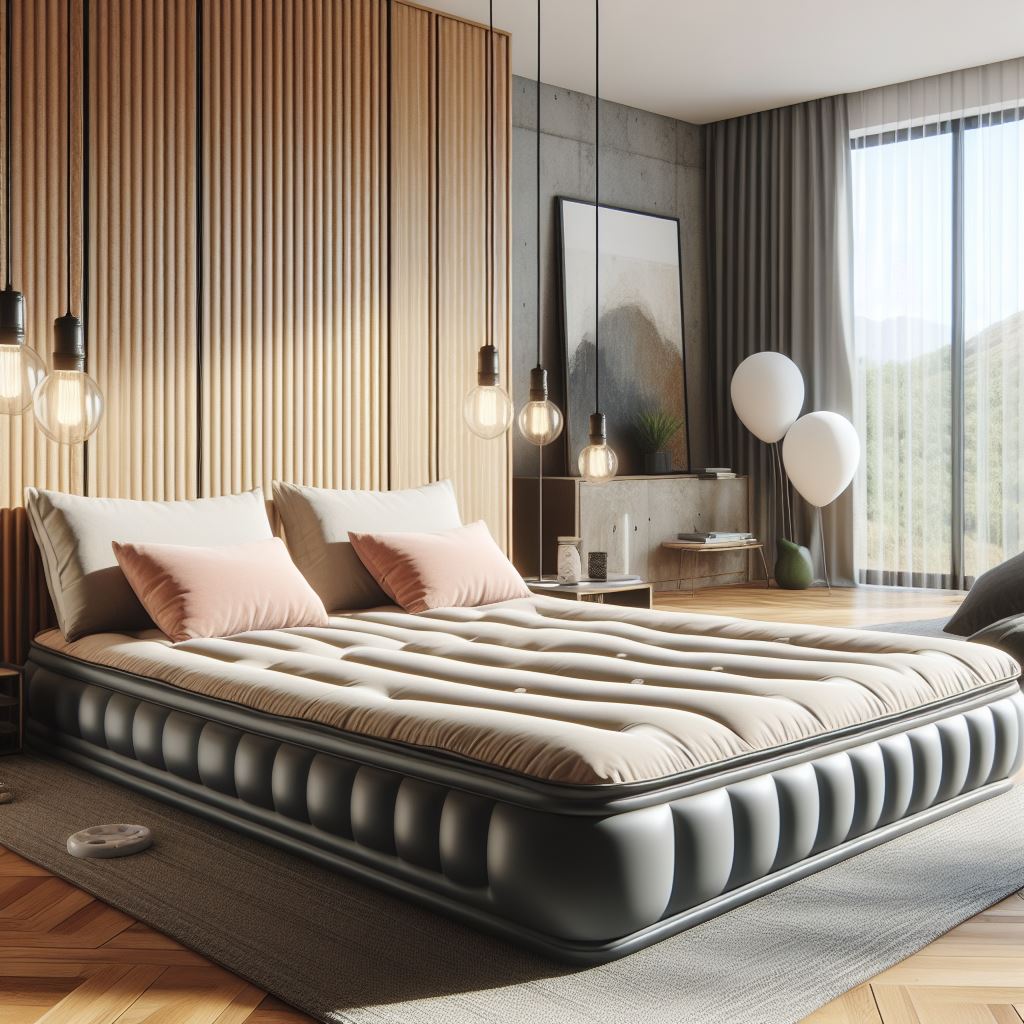The image showcases a contemporary, seemingly computer-generated bedroom, likely that of a fancy hotel or a wealthy individual. Dominating the scene is a large, air mattress-like bed, potentially a California king, with gray sides and a white surface, and adorned with two large white pillows and two smaller pink pillows. The bed sits on a gray rug laid over a light brown wooden floor. Behind the bed is a striking accent wall featuring gold-toned wood paneling with vertical strips interrupted by black sections, creating a modern aesthetic. The ceiling, approximately 16 feet high, supports various pendant lights hanging close to the bed, along with two slender, balloon-like lamps on the far left, and identical lamps on the right. A large sliding glass window adorned with thick gray curtains offers a view of grassy hills outside and serves as a backdrop for a small nightstand. The nightstand holds a green vase, a cup, and a painting, as well as a shelf for a phone. The window's sill is graced by two white balloons. A gray dresser situated nearby features another painting or mirror. The room, with its modern decor and intricate detailing, conveys a sense of luxury and meticulous design.